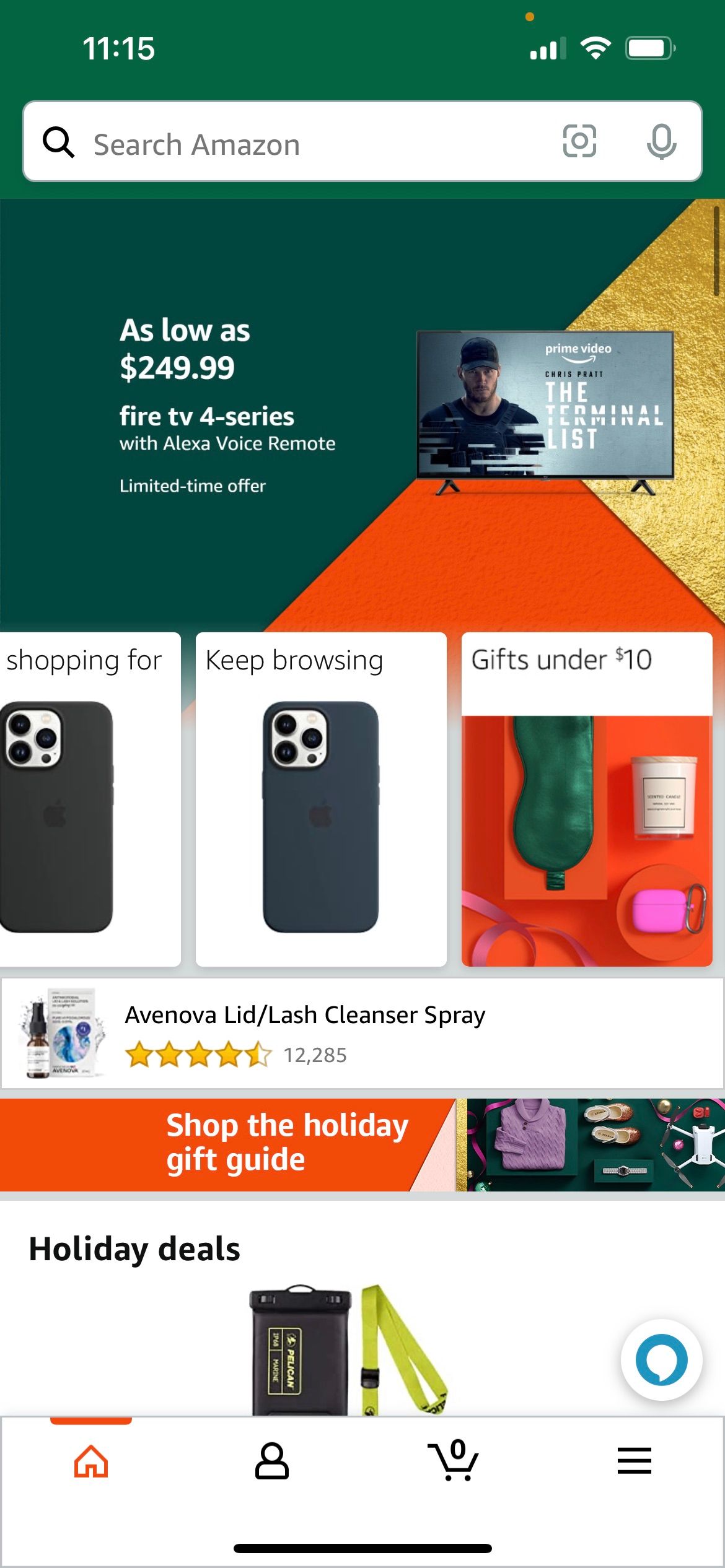The screenshot features a notification bar at the top displaying the time as 11:15 and a low battery warning. Below it, there's a promotion for a Fire TV 4-Series with Alexa Voice Remote, available for a limited time at $249.99. The screen is part of a shopping app, showcasing various sections like "Shopping for shows," "Keep browsing shows," and "iPhone gifts under $10." 

One highlighted product is Avanova Lid/Lash Cleanser Spray, which boasts a 4.5-star rating from 12,285 reviews. There are also links to the "Holiday Gift Guide" and "Holiday Deals." 

The layout includes a black bag with orange and green straps prominently displayed. Navigation icons at the bottom of the screen feature a home button, profile button, shopping cart, a three-line menu (often referred to as a "hamburger menu"), and a black chat bubble icon. Text is primarily in black, while the search bar at the top is white. The background is mostly white with accents of orange, green, and brown.